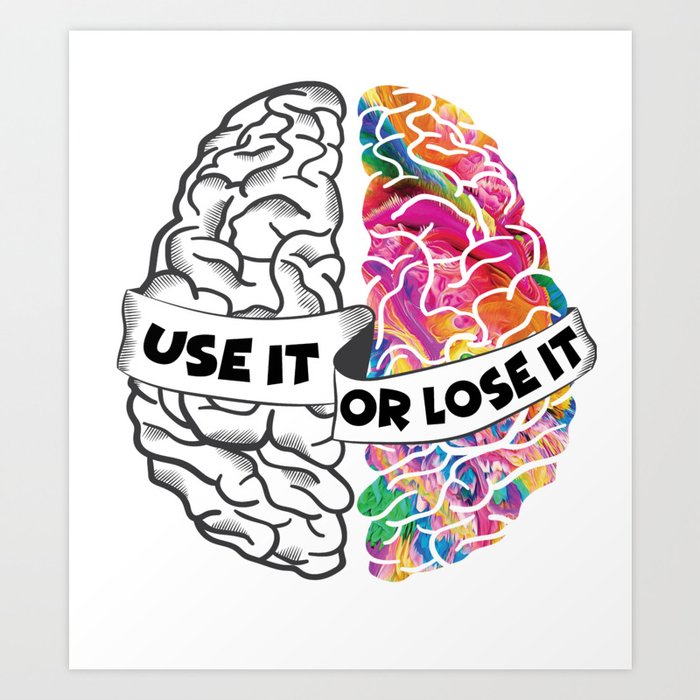This is an illustration of a human brain, split into two distinct halves. The left side of the brain is depicted in black and white with bold black outlines, while the right side bursts into a vivid spectrum of colors including pink, purple, blue, orange, yellow, red, green, bright blue, and lighter pink, all demarcated with bold white outlines. The background is white, matching the white wall it is displayed on. A prominent white banner with black text runs centrally across the brain image, proclaiming "USE IT OR LOSE IT". This phrase is split, with "USE IT" over the monochrome left half and "OR LOSE IT" over the colorful right half. The words are in large, slightly bubbled, capital letters. There is a clear space between the two brain halves, accentuating the division and the contrasting depictions of brain activity or usage.